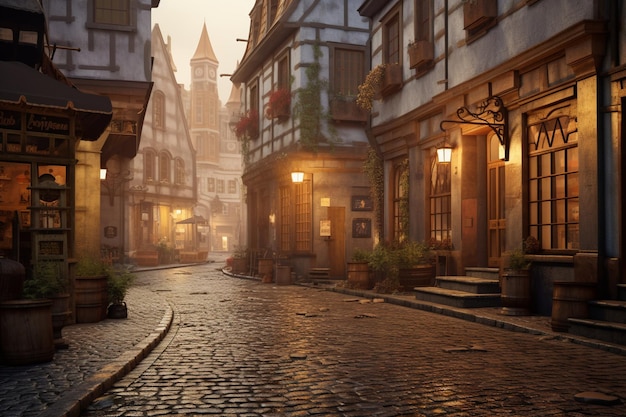This hyper-realistic painting portrays a winding cobblestone street through a small, Germanic-style medieval village. The cobblestone path starts at the bottom right and meanders out into the background, turning left before disappearing behind a building on the right. Flanking this street are white buildings adorned with brown latticework and windows. Green vines and red flowers climb the latticework, adding splashes of color to the scene. The first floors of these buildings, constructed of darker, wooden materials, suggest the presence of businesses, while the lighter, white-painted upper floors likely serve as lodging.

The setting appears to be at dawn or dusk, with a softly lit sky. Street lamps, emitting a warm orange glow, hang from the buildings, casting a comforting light over the cobblestone path. The windows of the buildings also exude a similar warm glow. On the left side, an open-faced building could serve as a gazebo or courtyard, contributing to the village’s quaint charm. In the distance, a clock tower rises at the end of the street, its pointed architecture echoing a more religious or imposing past. The vibrant greenery, meticulously detailed cobblestones, and the interplay of golden, ivory, and gray hues create a mesmerizing and nostalgic ambiance, hinting at both the bustling life and tranquil moments of this picturesque village.